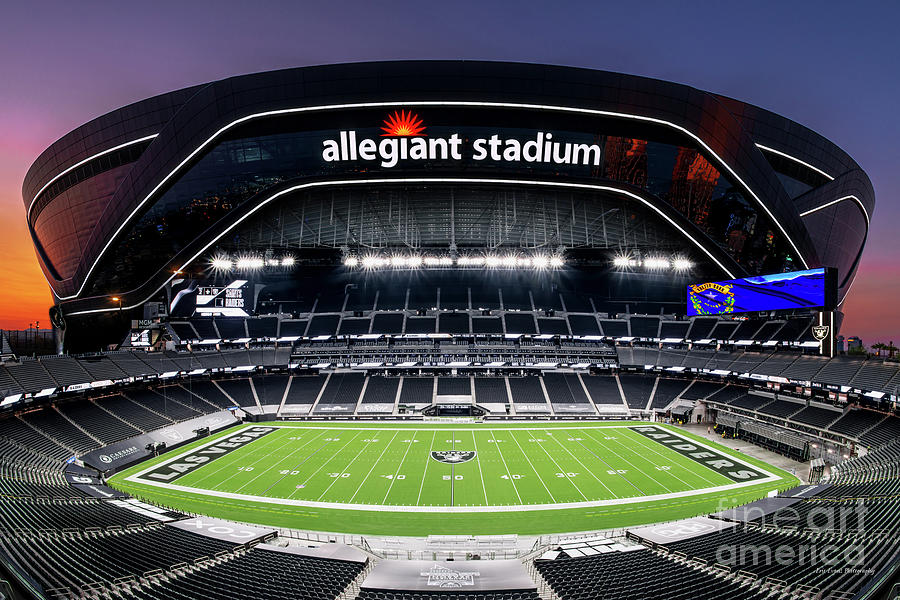The photograph showcases the stunning new Allegiant Stadium in Las Vegas, the future home of the Las Vegas Raiders. Captured during a striking sunset, the sky transitions from deep purples to vibrant oranges and reds, illuminating the distinctive black dome of the stadium. Clearly visible are the immense letters spelling out "Allegiant Stadium" atop the structure, with a sunrise logo over the "i." The perspective is from an elevated, somewhat external view, offering a comprehensive glance into the stadium’s interior. At its center is the pristine green football field, marked meticulously with yardage lines and numbers ranging from 10 to 50 across midfield. The end zones are emblazoned with "Las Vegas" on the left and "Raiders" on the right. 

Inside, the stadium’s impressive two tiers of seating are completely empty, though the area is brightly illuminated. A long, horizontal scoreboard stretches along the right side, displaying a blue image and an indistinct logo. Additionally, a second scoreboard on the right side prominently features the word "Raiders." A watermark from Fine Art America is discreetly placed in the lower-left corner of the image. The meticulous detail of this photograph beautifully captures both the grandeur and the tranquility of Allegiant Stadium in the serene evening light, highlighting its readiness to welcome fans for future events.